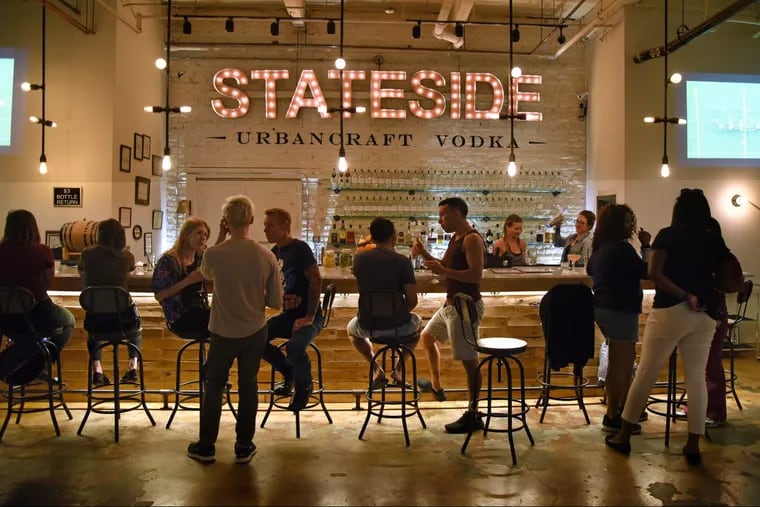The image captures an atmospheric and dimly lit bar featuring prominently displayed text reading "Stateside Urban Craft Vodka." The word "Stateside" is illuminated in red and white neon lights, while "Urban Craft Vodka" is boldly painted in black underneath. The background showcases four shelves stacked with an assortment of vodka bottles. 

In the foreground, a wooden bar runs horizontally across the image, with numerous bar stools occupied by patrons. Some individuals sit with their backs facing the viewer, while others are engaged in lively conversations, either standing or turned towards each other. To the right of the bar, two bartenders are at work. One, a woman wearing glasses, a green over shirt, and a darker undershirt, is shaking a cocktail shaker. 

The concrete floor spans the lower quarter of the image, and the white walls are adorned with various items including hanging pictures and a barrel in the top left corner. Overhead, eclectic light fixtures, comprised of bare bulbs and perpendicular extensions, illuminate the scene, enhancing the bar's inviting ambiance.